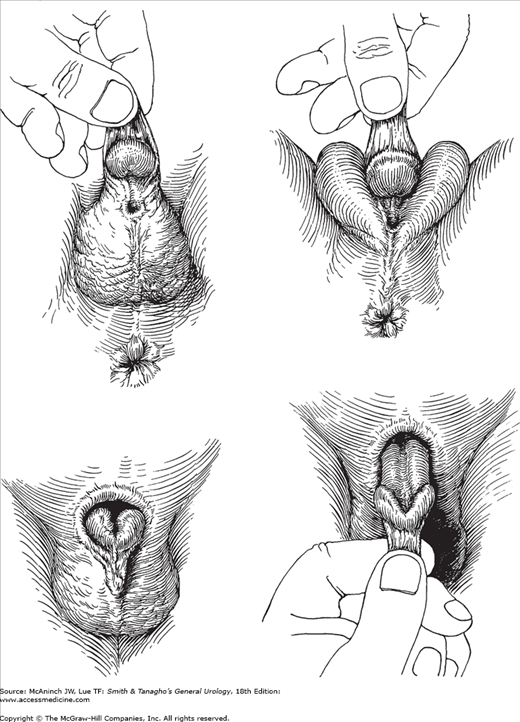This black and white anatomical illustration appears to come from an educational textbook on general urology. The image is divided into four sections, each depicting a human hand manipulating the genitalia to show different angles and details.

- **Upper Left:** A hand is holding the skin of a penis, exposing the testicles.
- **Upper Right:** Another illustration shows a different angle, resembling the labia or vaginal area.
- **Lower Left:** A close-up of the genitalia is shown without a hand, focusing on the anatomy.
- **Lower Right:** A hand pulls the skin again, presenting yet another view of the penis and surrounding area.

Small text in the lower left corner credits the source as "Mechanic JW2TF Smith and Tanago's General Urology, 18th Edition," and mentions www.accessmedicine.com and copyright by The McGraw-Hill Companies, Inc. All rights reserved. The precise text from the copyright is tiny and partially obscured in the illustration.